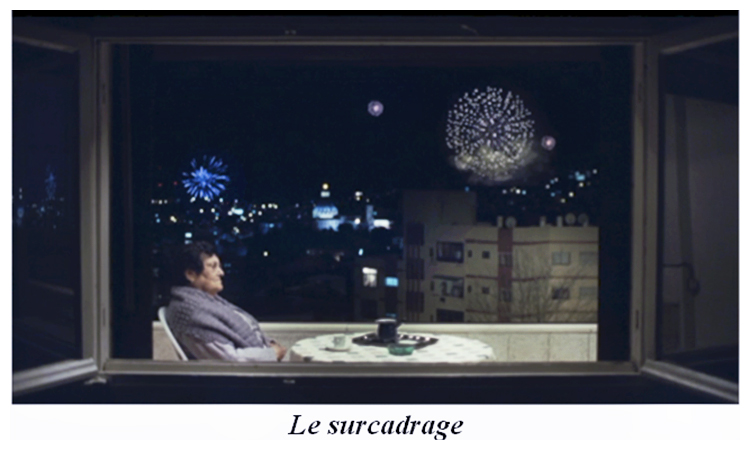The photograph depicts an androgynous-looking older individual with short black hair, seated at a round table covered with a white tablecloth. They are leaning back in a white chair, adorned in a gray, baggy garment with white sleeves, possibly draped with a blanket around the neck. The table features a black coffee pot and a white teacup, and the setting takes place on an outdoor balcony, indicated by the high vantage point overlooking multi-story buildings in the distance. It is nighttime, and vibrant fireworks light up the sky in hues of blue, light blue, and purple. The viewer's perspective is from behind a large plate glass window, and across the bottom of the image, text reads "Lee Sir Codridge" or a similar variation.